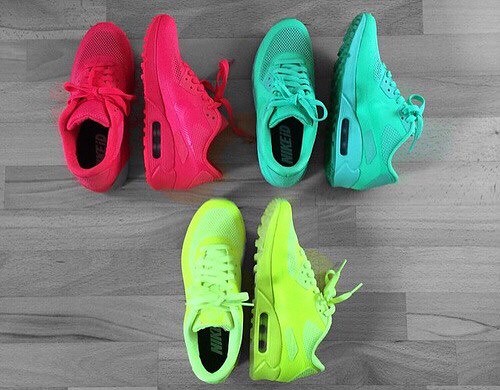This photograph depicts three pairs of identical athletic shoes, arranged for display on a dark gray hardwood floor. The photo is taken from an overhead perspective. In the top row, the pair on the left is a pinkish-red color, while the pair on the right is a light bluish-green. The single pair in the second row is bright yellow. Each pair of shoes consists of a left shoe positioned upright with the top facing up, allowing a view into the sole, and a right shoe lying on its side to show a side profile. All the shoes have tie-up laces that are neatly tied, feature black inner soles, and have a small black window toward the heel. These shoes appear to be brand new, likely displayed in a fashion typical for a retail sale.